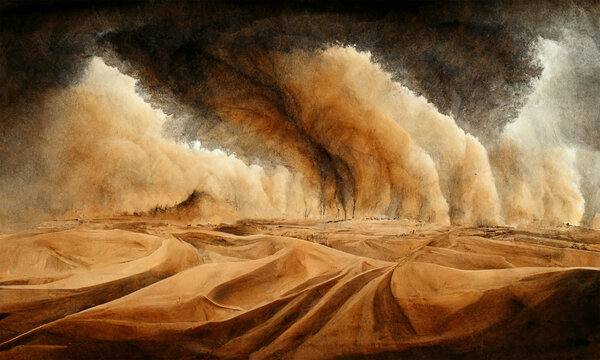The painting depicts a striking desert scene dominated by dark and earthy tones of white, black, brown, and tan. The foreground is filled with numerous sand dunes of varying heights and ridges, their medium brown color typical of desert sand. These dunes create an undulating landscape that stretches towards the horizon. Above, the scene grows more tumultuous; billows of sand and smoke seem to rush across the landscape, suggesting a powerful sandstorm in progress. The upper half of the painting is consumed by dark, ominous clouds, possibly storm clouds, that transition from lighter brown at their base to deep black at their peaks. The overall effect is a portrayal of a vast, open, yet perilous environment, where a significant, unsettling event disturbs the natural order.